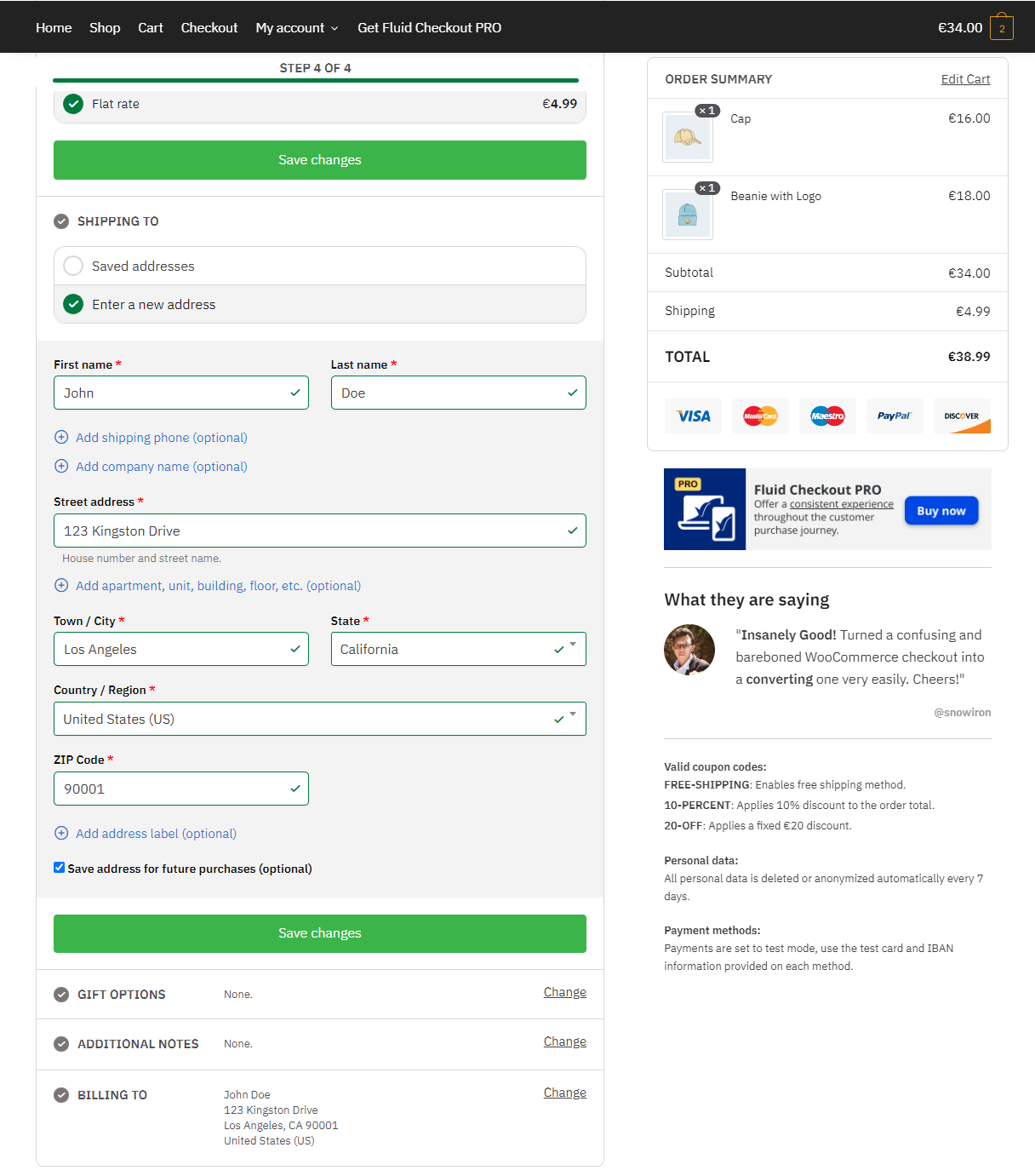The image is an online shopping checkout page with a structured and detailed layout. The header features a black banner with navigation options labeled: Home, Shop, Cart, Net, Checkout, My Account, Get Fluid, Checkout Pro, and a price indicator marked as €34. Two items are listed in the Shopping Cart.

On the left-hand side, a vertical navigation bar indicates that the user is on Step 4 of 4, named "Flat Rates," with a shipping cost of $4.99. Below this, a green button labeled "Save Changes" is prominently displayed.

The center panel of the page is dedicated to user input fields, all outlined in green. These fields prompt the user to enter their shipping information, including:
- First Name: John
- Last Name: Doe
- Phone (Optional)
- Company Name (Optional)
- Street Address: 123 Kingston Drive
- House Number and Street Number Name
- Apartment, Unit, Building, Floor, etc. (Optional)
- Town: Los Angeles
- State: California
- Country/Region: USA
- Zip Code: 9001

Additional fields allow the user to:
- Add an Address Label
- Save the Address for Future Purchases (this option is checked)
  
Beneath these fields, another green button labeled "Save Changes" is present. 

Further, the page shows sections for Gift Options and Additional Notes, both of which are marked as "None." 

Finally, the billing address is confirmed as the same as the shipping address, showing "E-Billing" details as "John Doe at the address above."